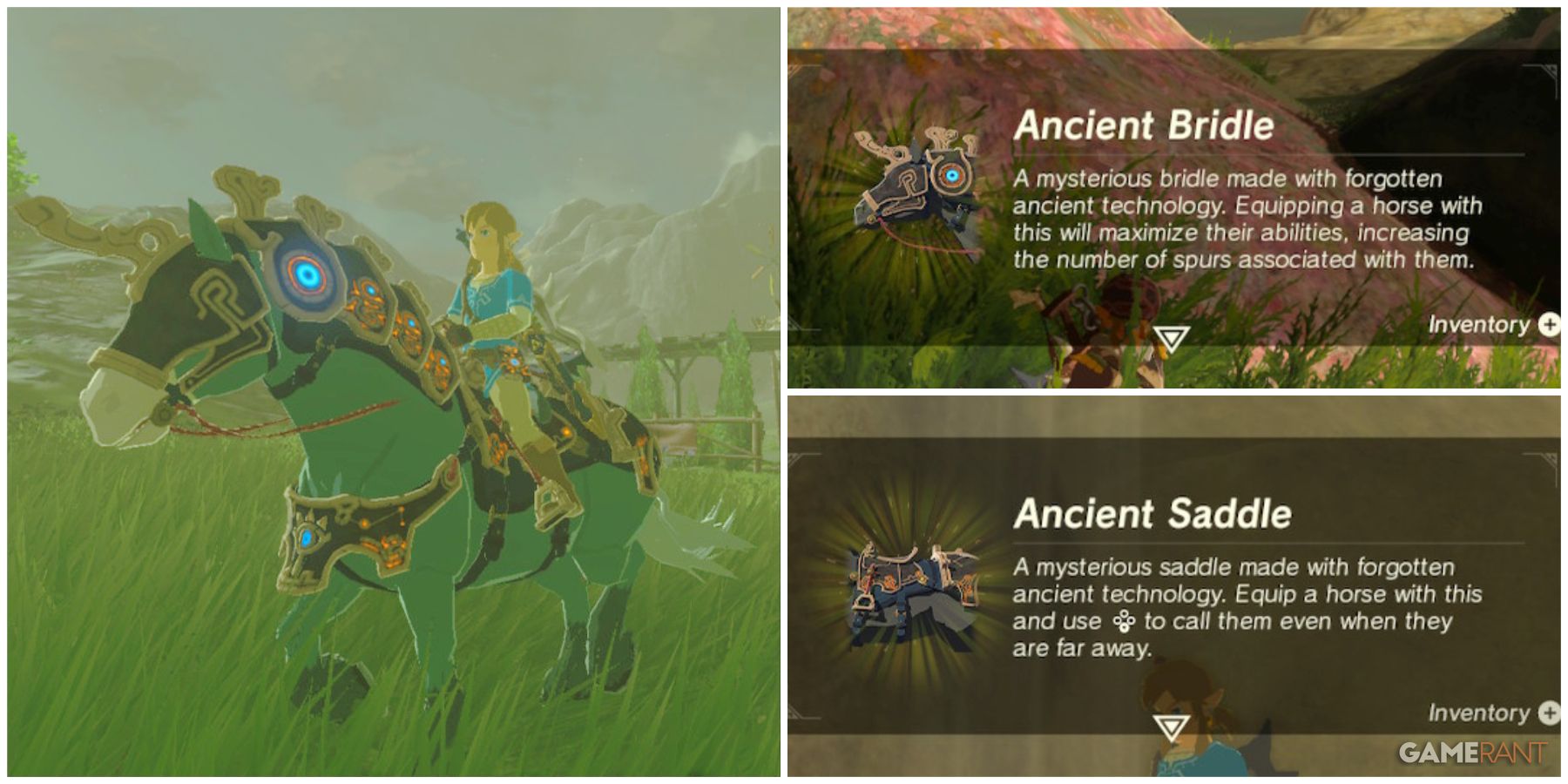The image is divided into three frames showcasing elements from a video game, likely "The Legend of Zelda." The left frame features a character, possibly Link, clad in a green shirt and brown pants, riding a green horse adorned with ornate, glowing armor. The armor covers the horse's head and neck, resembling ancient, mystical technology, with glowing lights and intricate designs that include gold-bordered saddles and a helmet with elaborate details. The scene is set in a lush, grassy field with towering mountains in the background, suggesting an expansive game environment. The horse appears vibrant and in motion, with its tail swishing behind.

The top right frame highlights an item named "Ancient Bridle," described as a mysterious bridle made with forgotten ancient technology that maximizes the horse's abilities, increasing the number of spurs the horse can use. This frame includes a close-up of the horse's head, overlaid on a backdrop of rolling hills.

The bottom right frame shows another item labeled "Ancient Saddle," similarly made with ancient technology. This saddle enables users to call their horse from afar using a game keypad. Both items emphasize their mystical and technological significance within the game's lore.

Overall, the scene intricately details the character and their horse, emphasizing the mythical elements of the game’s world through richly designed equipment and a picturesque, open-world setting.